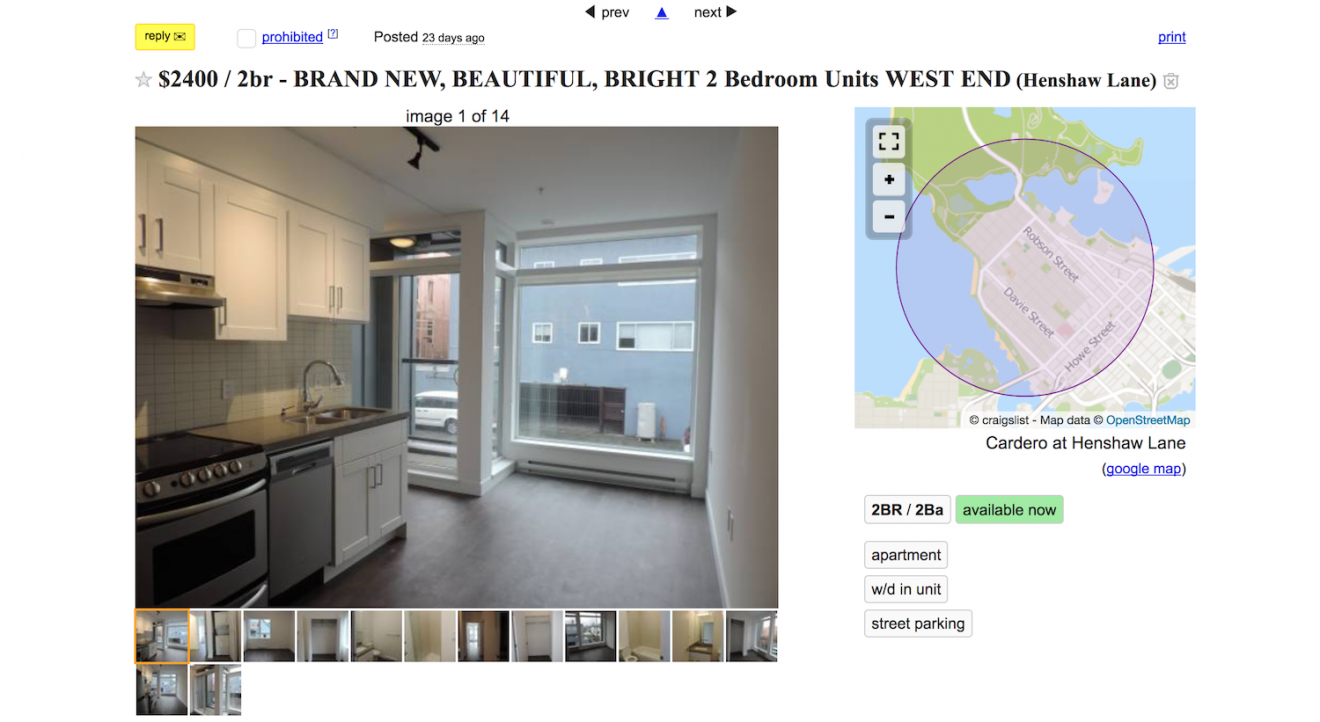Screenshot of a Craigslist website showcasing an apartment listing.

At the top center of the webpage, a navigation bar consists of three parts: a left-pointing triangle with the text "PREV" to its right, a blue triangle pointing upwards, and then the word "NEXT" in black followed by a right-pointing triangle. Just beneath this, on the next row, from left to right, is a black "REPLY" text over a yellow rectangular button, an unchecked blue link checkbox labeled "PROHIBITED," the text "posted 23 days ago," and a blue "print" link on the far right.

Below this row, the listing's header starts with a gray, unhighlighted star, followed by the price "$2400" and "2BR - BRAND NEW BEAUTIFUL BRIGHT 2" in capital letters. The text "bedroom units" follows in title case, then "West End" in capital letters with "Henshaw Lane" in parentheses. A trash can icon is to the right of this information.

The main content of the listing is divided into two sections: the primary content on the left and the sidebar on the right. On the left, there is an "Image 1 of 14" indicator. The current image displayed is of a modern, clean, and updated kitchen area with no furniture, featuring white upper and lower cabinets, a dishwasher, and a sink. The 13 other images are available as thumbnails below this larger image.

On the right, the sidebar section starts with a square map preview that includes map navigation icons, such as zoom in and out. The map features a purple circle with a light purple overlay indicating the apartment's location. At the bottom right corner of the map, the label "Craigslist map data" is visible, confirming this is indeed a Craigslist page. Below the map preview, the address "Cardero at Henshaw Lane" is provided, followed by a clickable "Google map" blue link in parentheses.

Additional listing details are displayed below: "2BR / 2BA" in light gray with a gray outline, "available now" in black text on a green background, and other details like "apartment," "WDN unit," and "street parking" within rectangular outlines. The background for these details is white.